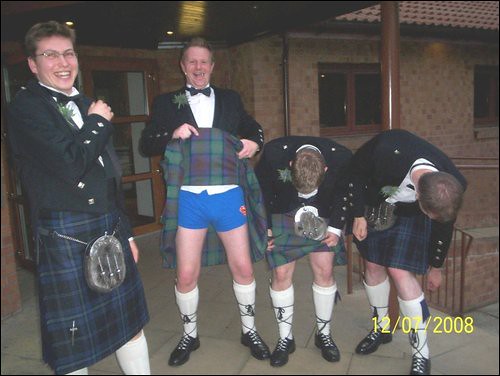The photograph captures four white men at what appears to be a jovial pre-wedding moment, as suggested by their attire and surroundings. Each man is dressed in a blend of traditional and formal wear: black tuxedo jackets with white undershirts and black bow ties on top, paired with kilts and knee-high white socks crisscrossed with black strings, along with black dress shoes sporting white laces. The two men in the center wear kilts with purple and green squares, while those on the outer sides don kilts with blue and black squares. They stand in front of a brick building that resembles a church, featuring visible windows and a door, indicating they might be preparing to go inside. The light-hearted spirit is evident as the two men on the right lean down, possibly adjusting their kilts or socks, exposing blue shorts and the tucked-in bottom of a white shirt on one of them. Meanwhile, the men on the left are captured laughing and smiling. A yellow date stamp at the bottom right corner of the image reads "12/07/2008," marking this cheerful moment in time.